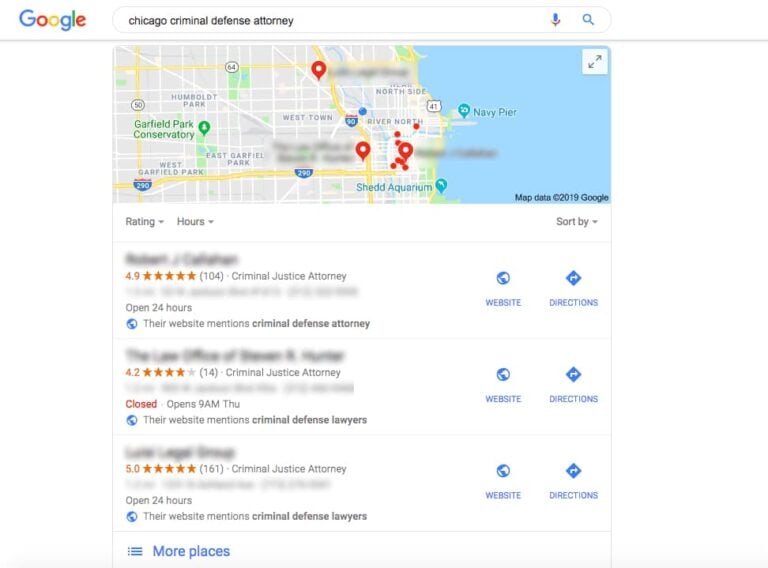The screenshot is taken from Google Maps, displaying a search for "Chicago criminal defense attorney" in the search bar. The interface appears to be from a desktop or mobile application. On the left, the familiar Google logo is visible in its iconic colors: blue, red, yellow, blue, green, and red. Beneath the logo, the white search bar contains the query with a black text and is accompanied by a blue microphone icon for voice search and a blue magnifying glass icon for initiating the search.

To the right is a map of Chicago, prominently featuring Lake Michigan in blue. Newport Pier, which extends into the lake, is also marked in blue. The city's geography is primarily shown in shades of gray, indicating urban areas. Green spaces, representing parks, are sporadically located mostly on the left side. 

The map also contains a network of streets, illustrated in white, running north-south and east-west. Larger roadways, likely major interstates and highways, are highlighted in white and yellow. Various markers on the map are red, though the names of specific locations have been blurred out. 

Below the map, three businesses related to the search term are listed, each with their ratings partially redacted. The visible ratings are 4.9, 4.2, and a perfect 5.0. On the right side of each listing, there are two blue icons: one for the website (depicted by a globe) and another for directions (represented by a white arrow within a blue circle).